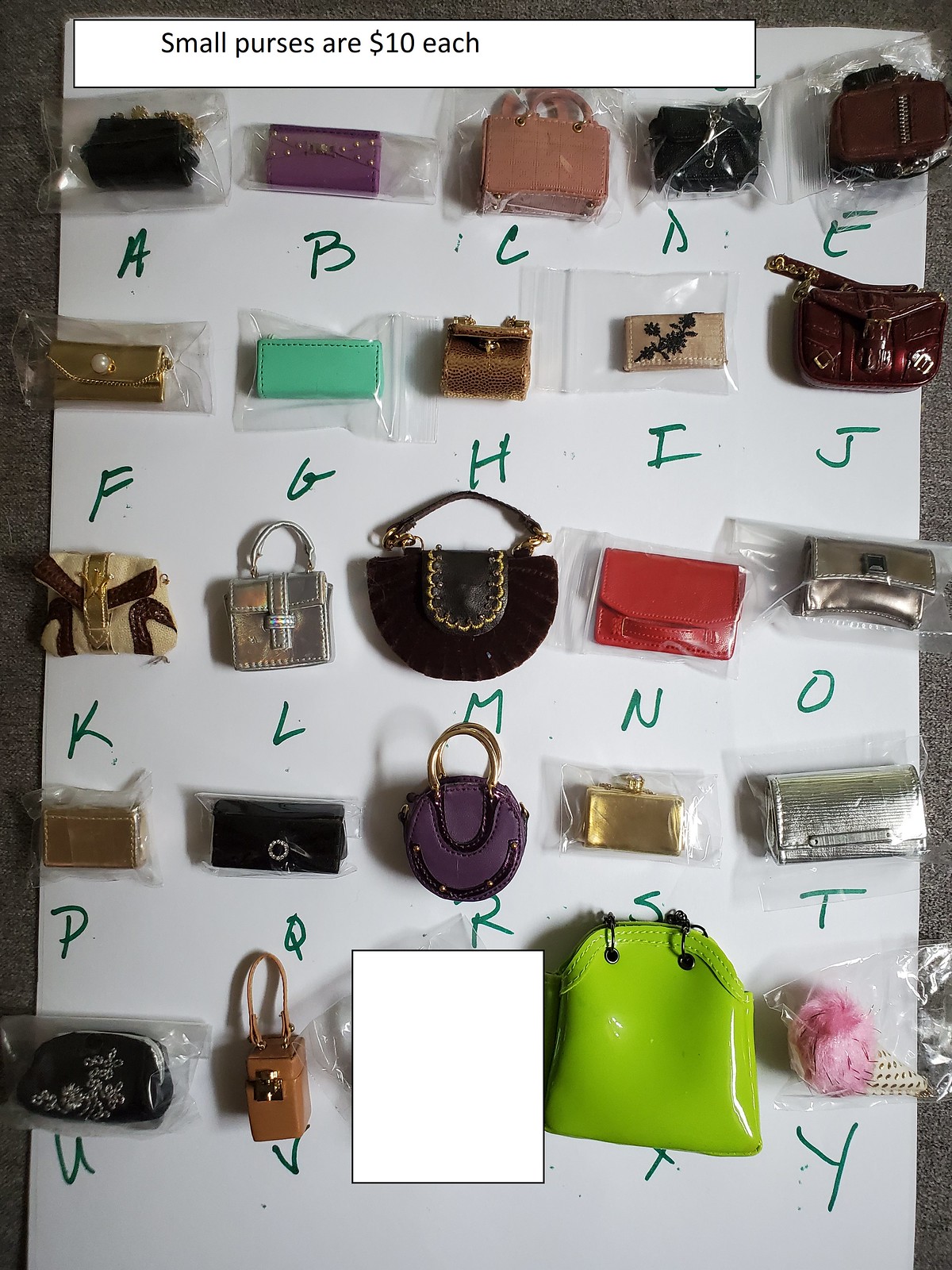This image showcases an organized display of small purses mounted on a large white backer board. Each purse is encased in cellophane and is accompanied by a handwritten letter ranging from A to Y, with the exception of W, which is obscured by a white symbol. The purses, available for $10 each as indicated by the sign at the top, exhibit a variety of colors and designs. These include vibrant shades like neon green, red, and light blue, as well as classic tones such as black, silver, and brown. The purses come in diverse styles—some are miniature handbags with large straps, others have the classic rounded purse straps, and a few are shaped like billfold pouches. Notably, there is a pink fuzzy purse shaped like an ice cream cone. The display is neat, with the purses arranged in rows and labeled in green marker, emphasizing both functionality and visual appeal.